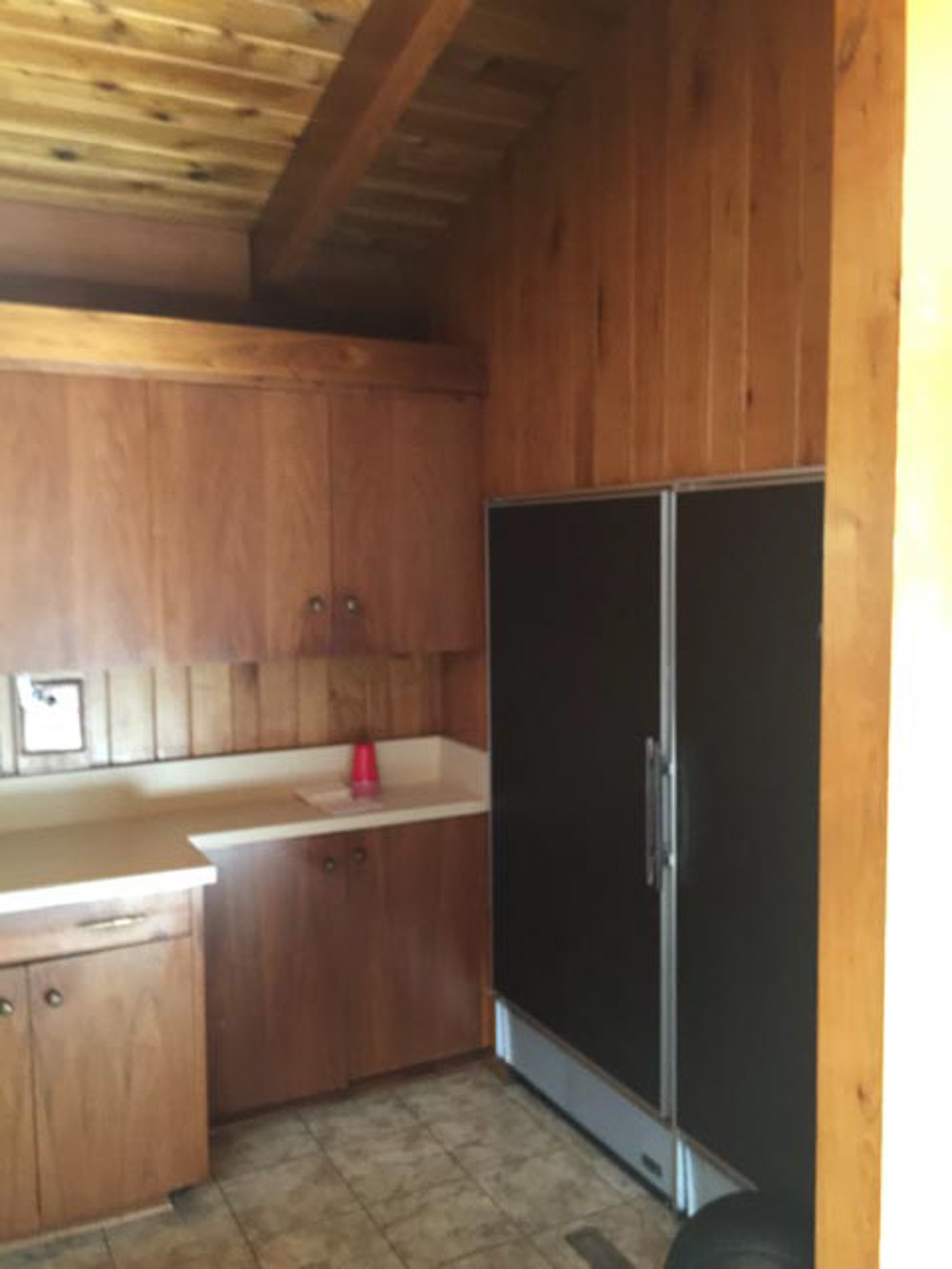The photograph depicts a vintage-style kitchen characterized by an abundance of wood elements. The walls are paneled in a dark or golden brown wood, giving the space a rustic charm. The ceiling features exposed beams in a lighter wood, creating a pleasing contrast with the walls. Dominating the scene are wooden cabinets, both above and below the beige granite countertops, with black, round ball-shaped handles.

The flooring is a textured gray tile with darker gray patterns, adding depth to the room. A red solo cup sits prominently on the countertop. Situated towards the right side of the image, a large black and silver double-door refrigerator is built into the wall, flanked by a black flip-top trash can. The refrigerator is accentuated by its sleek silver handles and trim.

Above the refrigerator and along the walls, the wood paneling continues, seamlessly integrating with the overall design. The room also features a beige marble-type floor. Socket paneling is visible underneath the cabinets, where a few red cups are stored upside down. This kitchen combines practicality with a nostalgic aesthetic, emphasized by its meticulous woodwork and thoughtful details.